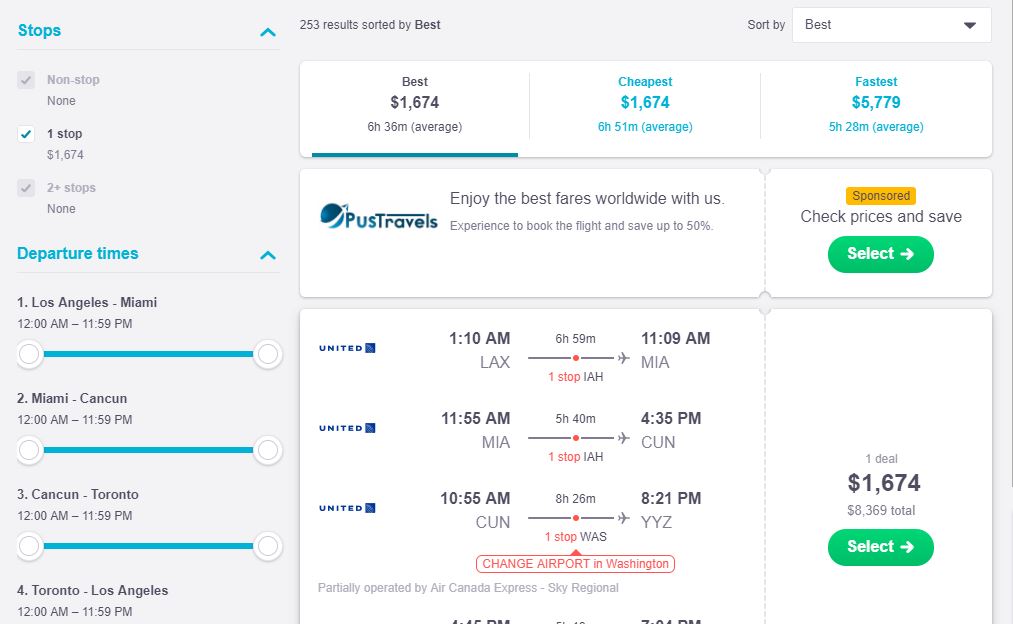The image displays a meticulously organized flight search results page featuring 253 results, sorted by "Best." It highlights various flight options with a blue checkmark indicating the selection of one-stop flights against non-stop and two-plus-stop options, which remain unselected in gray. The departure times are listed comprehensively:
1. Los Angeles to Miami (12:00 a.m. to 11:59 p.m.).
2. Miami to Cancun (12:00 a.m. to 11:59 p.m.).
3. Cancun to Toronto (12:00 a.m. to 11:59 p.m.).
4. Toronto to Los Angeles (12:00 a.m. to 11:59 p.m.).

The "Best" flight option features an average duration of 6 hours and 36 minutes, detailed as "6H 36M." There are also indications of the "Cheapest" flight at 6 hours and 51 minutes, and the "Fastest" flight at 5 hours and 28 minutes, offered at a higher fare of 5,779. A promotional banner invites travelers to enjoy the best fares worldwide, highlighting the ability to book flights and save up to 50%.